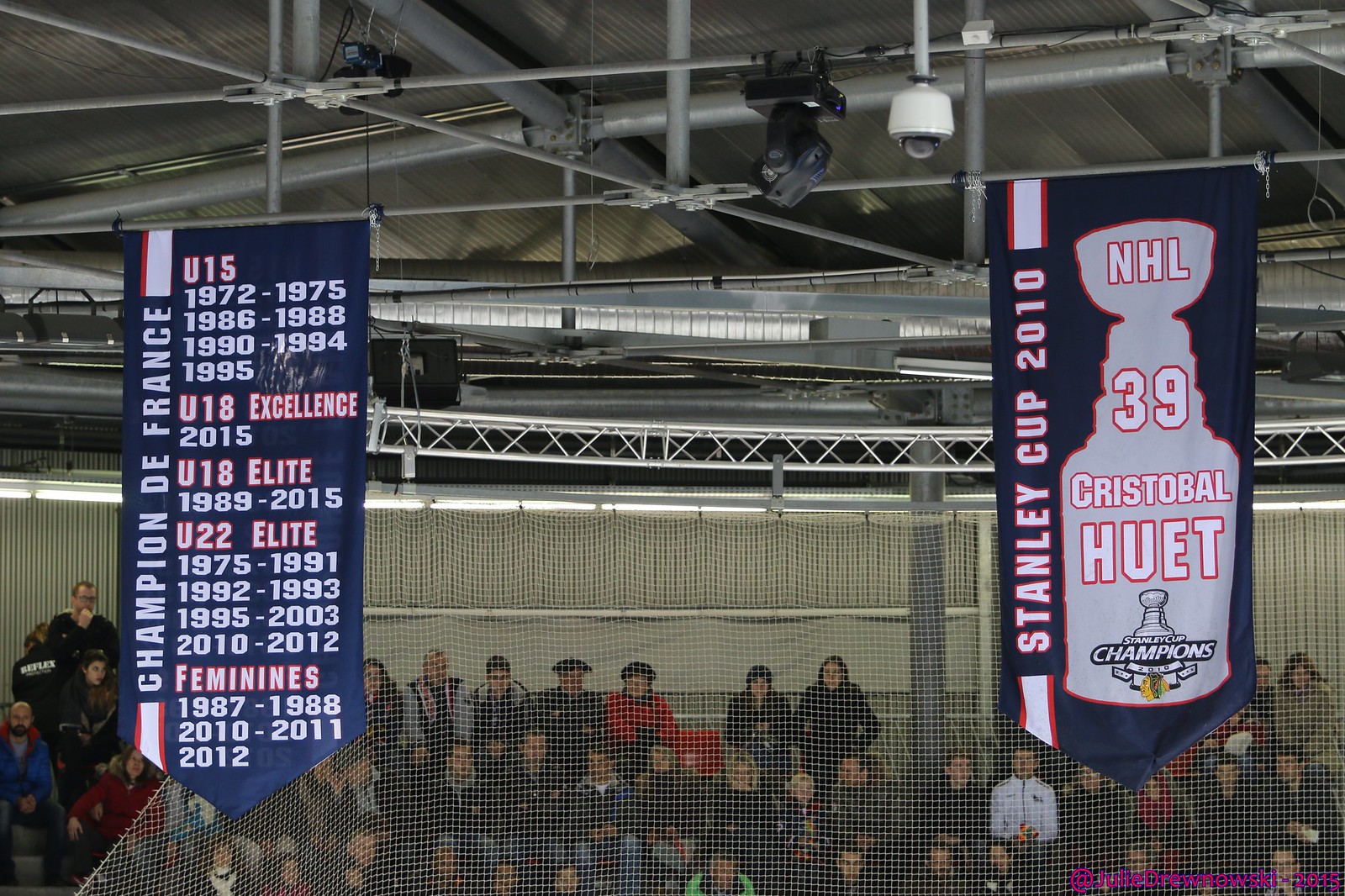This detailed image captures an indoor arena, possibly an ice hockey rink, filled with spectators seated in the stadium seats behind a protective net. The ceiling, structured with metal beams, prominently displays two significant banners. On the left hangs a blue banner, adorned with multiple chronological achievements: "Champion de France" detailing various team accolades such as "U15: 1972-1975, 1986-1989, 1990-1994, 1995," "U18 Excellence: 2015," "U18 Elite: 1989-2015," "UTT Elite: 1975-1999, 1992-1993, 1995-2003, 2010-2012," and "Feminines: 1987-1988, 2010-2011, 2012." On the right, another blue banner features a gray depiction of the Stanley Cup trophy and includes inscriptions like "Stanley Cup 2010," "NHL 39," and "Cristobal Hewitt Championship." The photo elucidates a vibrant, indoor sporting environment festooned with the celebratory history of the arena, painting a vivid picture of its storied past and its commitment to excellence across various levels and categories of the sport.